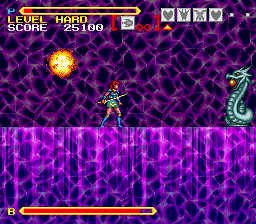The image is a detailed screenshot from a two-dimensional pixel art video game. At the center, a warrior with long red hair stands poised, wearing a blue dress and matching knee-high boots with orange knee guards. In her right hand, she wields a sword. To her right, a menacing green dragon stands upright, its head adorned with spikes and emitting a fiery barrage. The game setting features a horizontal playing field across the bottom, colored in varying shades of purple with dark blue and black mixed in. The upper background is predominantly black, interwoven with dark purple web-like textures. Bright details of the game overlay are visible: the yellow level indicator and the word "hard", a score of 25,100 in white, and four gray box icons—two hearts and two X's. A horizontal rectangular gauge at the bottom, featuring a red-orange line and the letter "B" in yellow, indicates minimal player progression. The entire scene is imbued with a purple haze, adding a mystical ambiance to the battle.